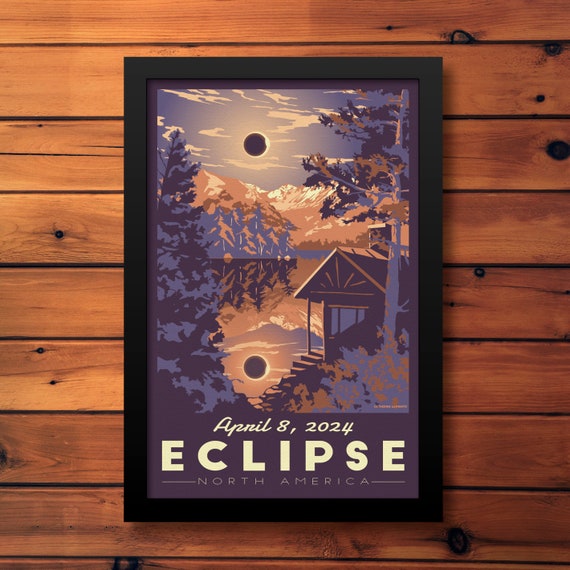The detailed image is of a framed poster hanging on a medium-brown, wooden plank wall, rich with knot holes, creating a rustic backdrop. The poster is encased in a simple, black wooden frame. The artwork within depicts a serene, dusk-like scene in hues of blue, purple, and occasional pink or brown tones. It features a small cabin nestled in a forest with trees of brown and blue around a central lake. Above, the sky is depicted with wispy clouds and a dark, purplish-blue gradient, dramatically showcasing a solar eclipse occurring on April 8, 2024. The sun is nearly obscured by the moon, leaving only a bright halo visible, which is also reflected in the calm waters of the lake below. The bottom of the poster is inscribed with "April 8, 2024, Eclipse, North America," anchoring this ethereal scene to a specific moment in time.